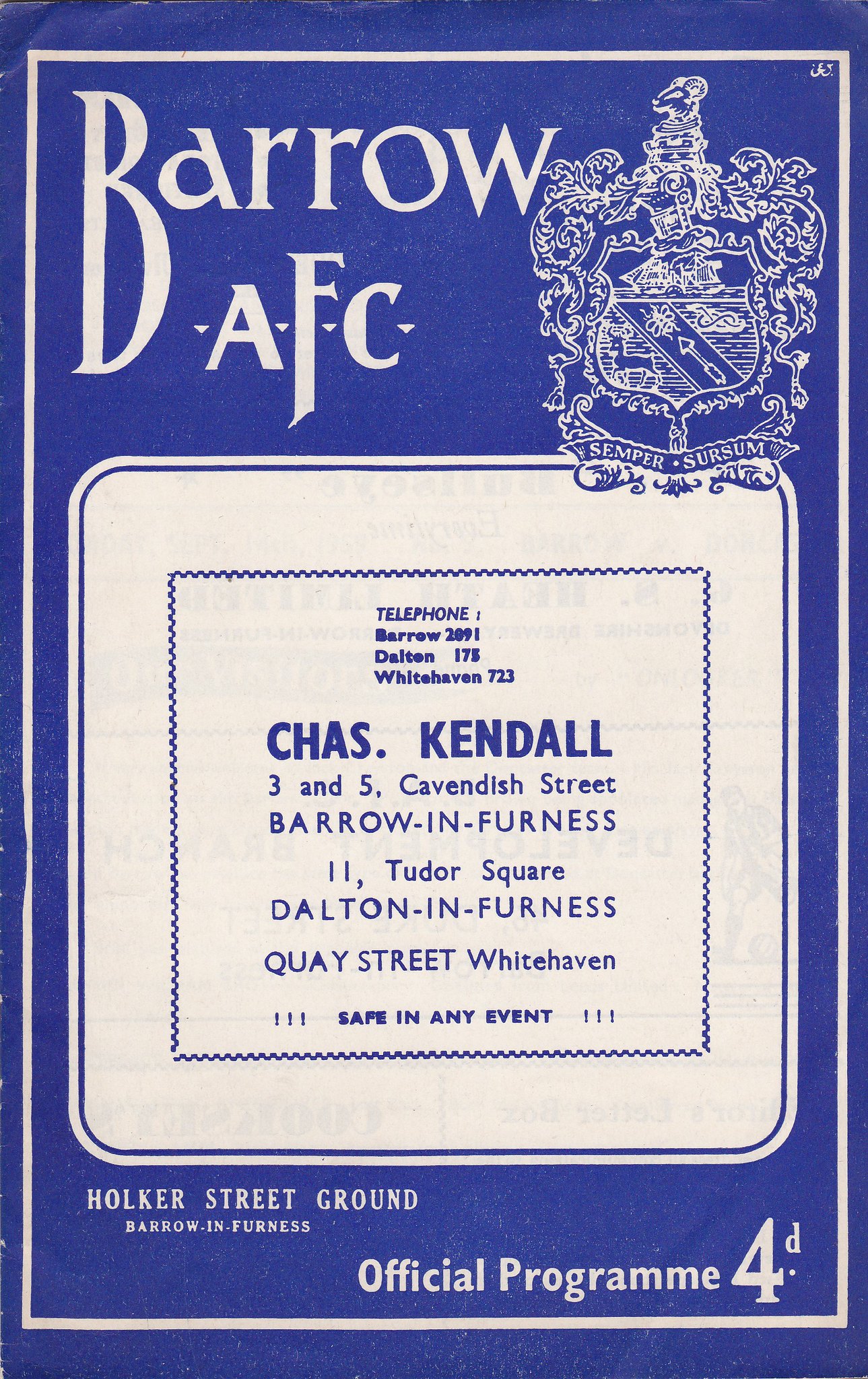The cover of this official program features a predominantly blue and white color scheme. The background is blue, framed by a thin white border. At the top left, the program title reads "Barrow AFC" in large, white letters with a distinctive stylization of "A*F*C," where the "F" resembles an elongated sword. Adjacent to this, on the right, is the Barrow AFC emblem depicted as a white shield adorned with decorative elements.

Centrally, there is a white, rounded rectangle bordered twice by blue lines. This section appears to highlight an advertisement for Chaz Kendall, listing multiple addresses as follows: "3 and 5 Cavendish Street, Barrow-in-Furness"; "11 Tudor Square, Dalton-in-Furness"; and "Quay Street, Whitehaven." Below this, the phrase "safe in any event" is noted in small print.

Towards the bottom of the cover, "Holker Street Ground" is displayed in white letters against the blue background, with "Barrow-in-Furness" specified beneath it. The bottom section states "Official Program" in mixed case, ending with "4-D," possibly indicating the program's price. The top left corner of the cover is slightly bent, adding a touch of authenticity to this vintage program design.